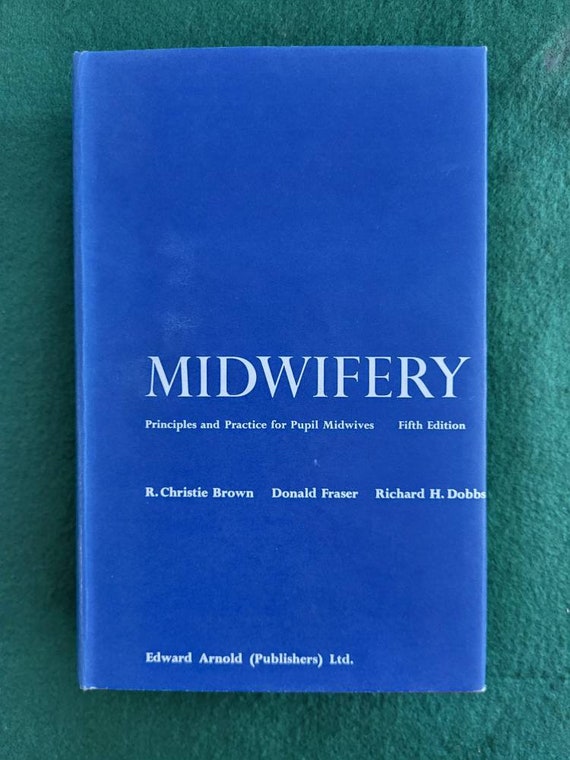The image features a photograph of an aged blue book titled "Midwifery," prominently displayed in white text. "Midwifery" is the largest text on the cover, while beneath it, in significantly smaller font, it reads: "Principles and Practice for Pupil Midwives, 5th Edition." Below this, the authors are listed as "R. Christie Brown, Donald Fraser, Richard H. Dobbs." Near the bottom of the cover, it states "Edward Arnold Publishers Ltd." The book's cobalt blue cover has worn edges, suggesting it has been well-used and cherished. The book rests on a slightly textured green background, which appears to be made of leather or suede, adding a subtle contrast to the blue cover.